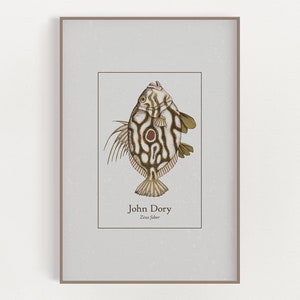This is an image of a framed drawing of a fish, featured as an artwork hanging on a white wall. The artwork is encased in a thin, gold or brown-colored frame with a white border. Depicted vertically, the fish's head is at the top and its tail is at the bottom. The monochrome drawing, primarily black and white, showcases intricate details: veiny patterns ripple from head to tail, forming a striking visual tapestry. Spiky dorsal fins add texture, while a prominent pinkish circle centered on its body resembles an eye. Below the fish, the name "John Dory" is inscribed, attributing the artwork to the artist.